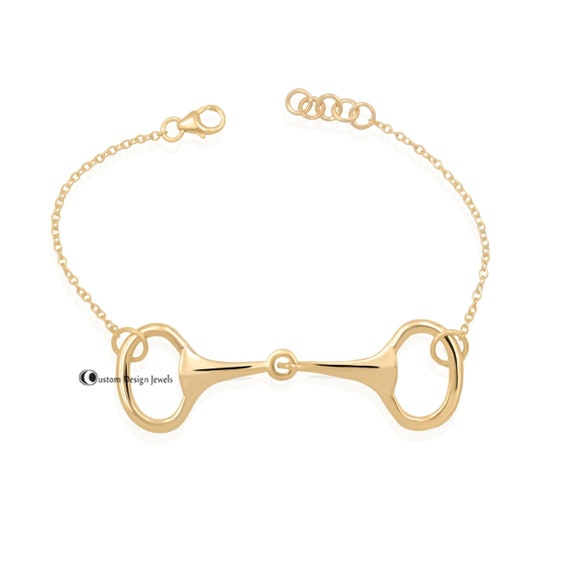This is a detailed image of a yellow gold bracelet against a clean white background. The bracelet features a central design comprised of two interlocking circles connected by a horizontal bar, with a round open circle in the middle acting as an additional connector. Attached to each of the two outer circles is a delicate gold chain made up of small interlinked rings. The bracelet is displayed unclasped, with a visible clasp on one end and small connecting hoops on the other. In the lower left corner, there is the black text "Custom Design Jewels," with the "C" stylized as a prominent black and white logo.